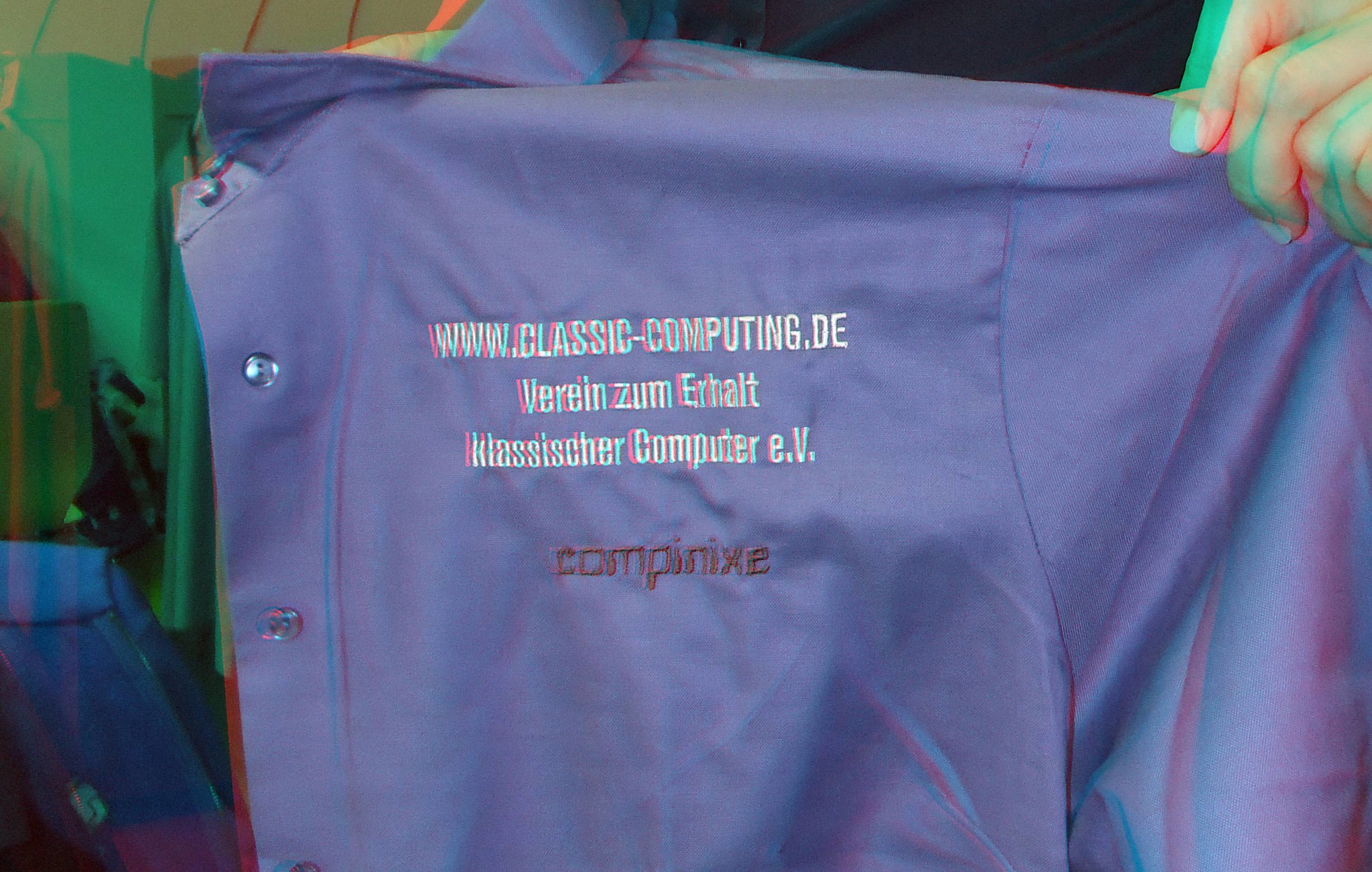This color photograph, taken indoors, captures a person holding up a light blue, button-down work shirt. The shirt, which features buttons down the front and on the sleeve cuffs, bears embroidered text in white reading "www.classic-computing.de" along with "Verizon, Earhart, Classiker, Computer, EV." Additional text in a dark, almost purple color reads "cam pan X." Visible in the image are the person's hands with three fingers gripping the shirt in the upper right corner and possibly a finger on the left. The background includes a green and white striped pattern, a piece of green fabric, and some grayish-brown material, all adding to the indoor setting.